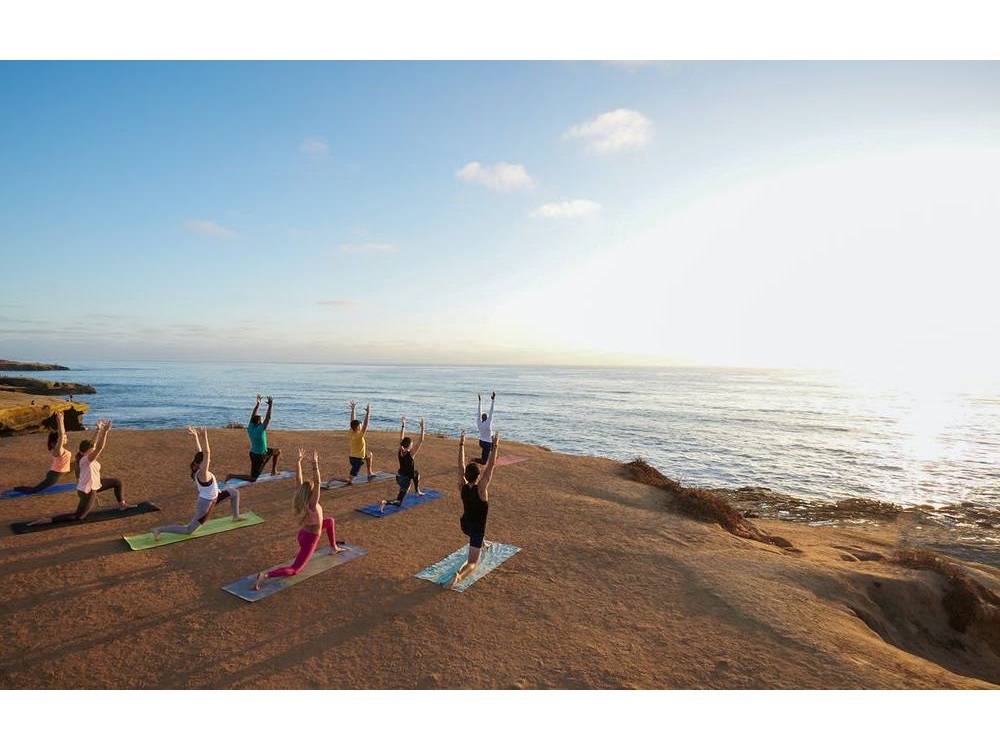This image captures a group of people engaging in a yoga session on a beach hillside with a stunning ocean view in the background. The scene is bathed in the dramatic light of a setting sun, casting long shadows behind the participants and illuminating the sky in hues of blue with scattered clouds. The group, consisting of predominantly women with at least one young black man, is positioned on brightly colored mats—including royal blue, lime green, gray, black, light blue, turquoise, and coral—spread out on the sandy and slightly rocky terrain that features sparse vegetation. Attired in a variety of exercise clothing in colors like black, yellow, pink, green, orange, white, and gray, they are in a half-kneeling, half-genuflecting pose with arms raised towards the sun. The deep sandy color of the beach contrasts with the grayish-blue ocean and the gradations in the sky, which transition from medium blue to nearly white where the sun’s rays are strongest.